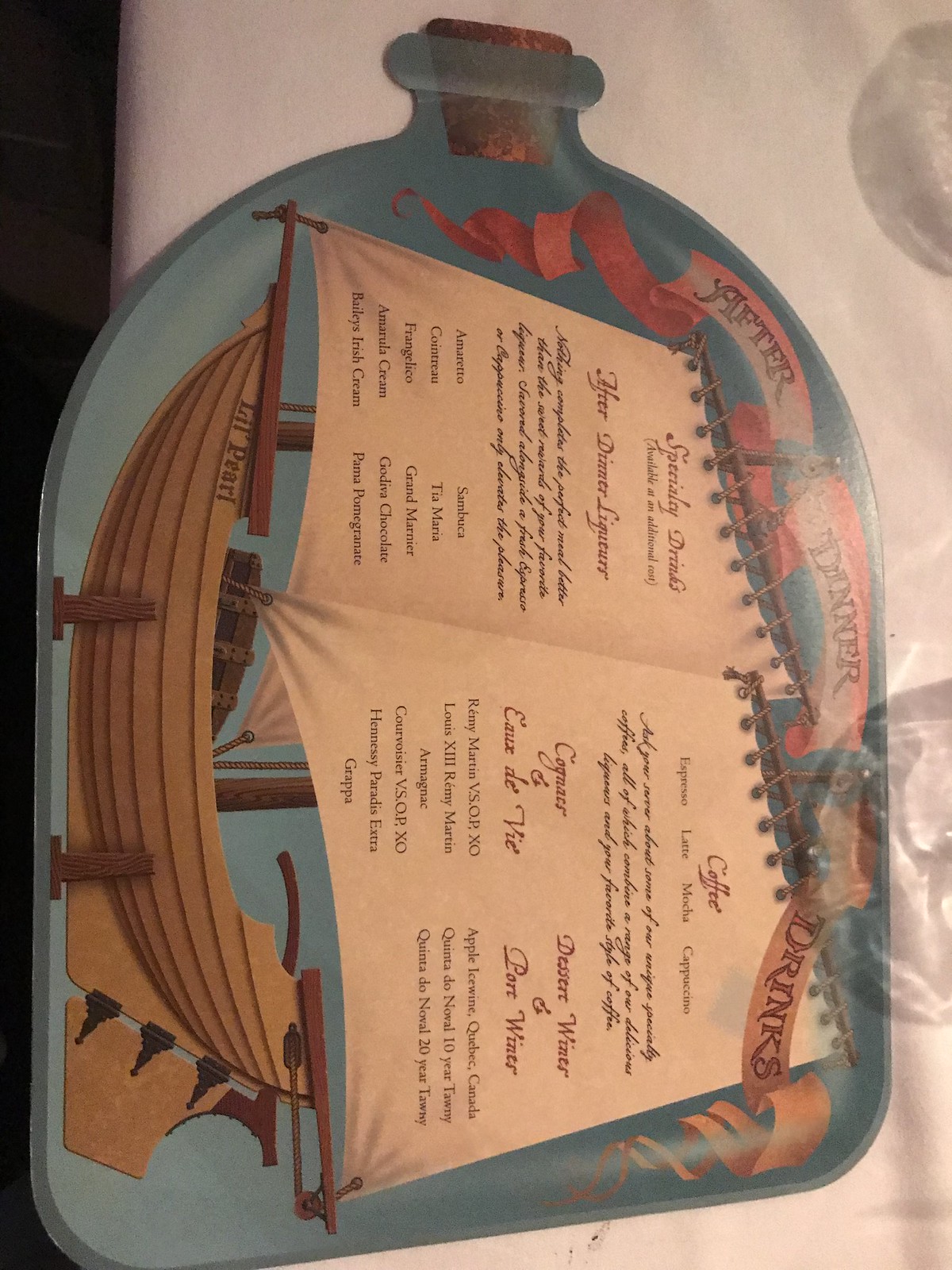This image features a creatively designed restaurant menu that has been photographed in a vertical portrait orientation, despite the original horizontal layout being rotated 90 degrees to the right. This unique presentation adds to the menu's charm, although it does make it more challenging to read. 

The menu itself is illustrated on the sails of a ship, which are positioned within a vertically-oriented, corked bottle—a classic "ship in a bottle" concept. The bottle is depicted with a striking blue color and a brown cork sealing its top. It's a notably wide bottle set against a blue background.

Inside the bottle, the ship is intricately illustrated, with its white sails adorned with vibrant red text listing the menu items, and black text providing descriptions. The ship, named "Little Pearl," is rendered in brown and features a prominent scrolling banner above its sails. The sails are fastened to the mast in a spiral notebook format, secured by numerous hooks, adding a whimsical touch to the design.